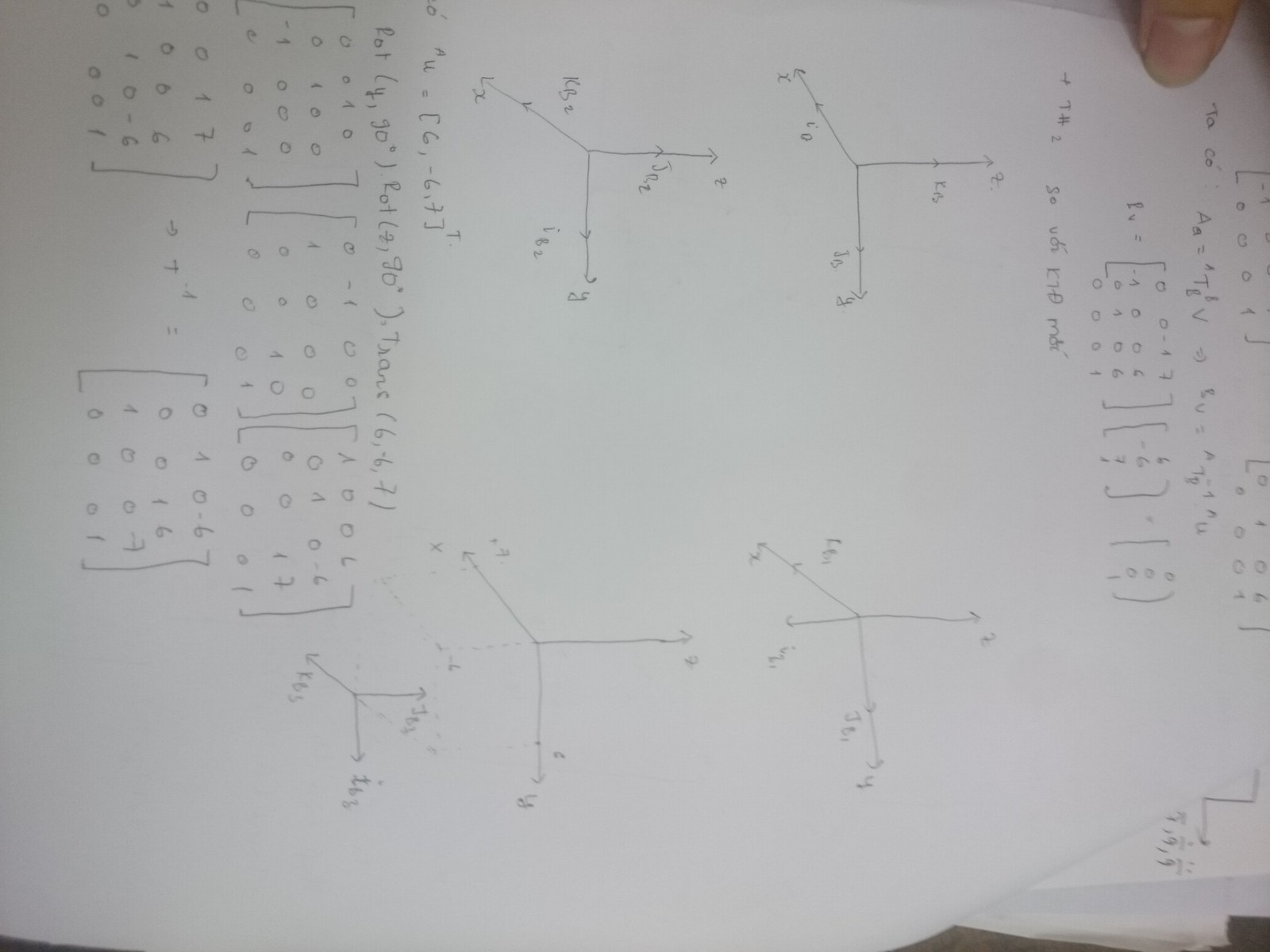A slightly wrinkled white piece of paper filled with dense scientific writing is presented sideways, making it somewhat challenging to decipher. At the top of the page, the text reads "T-O-C-O" followed by "Aa = TGV." Below this heading, there's a scattered series of numbers, starting with "1" and then followed by "0, 0 - 1, 7." The paper is populated with various sets of numbers enclosed in brackets, such as "4006, 0406, 0001, 6671," with each set varying in length. There are also at least five small diagrams featuring X and Y axes, although the measurements and graphs remain unclear. Additionally, there's a notable bracketed set containing "6, -6, 7." The page is cluttered with multiple mathematical equations featuring parentheses, creating a complex and somewhat baffling array of information.